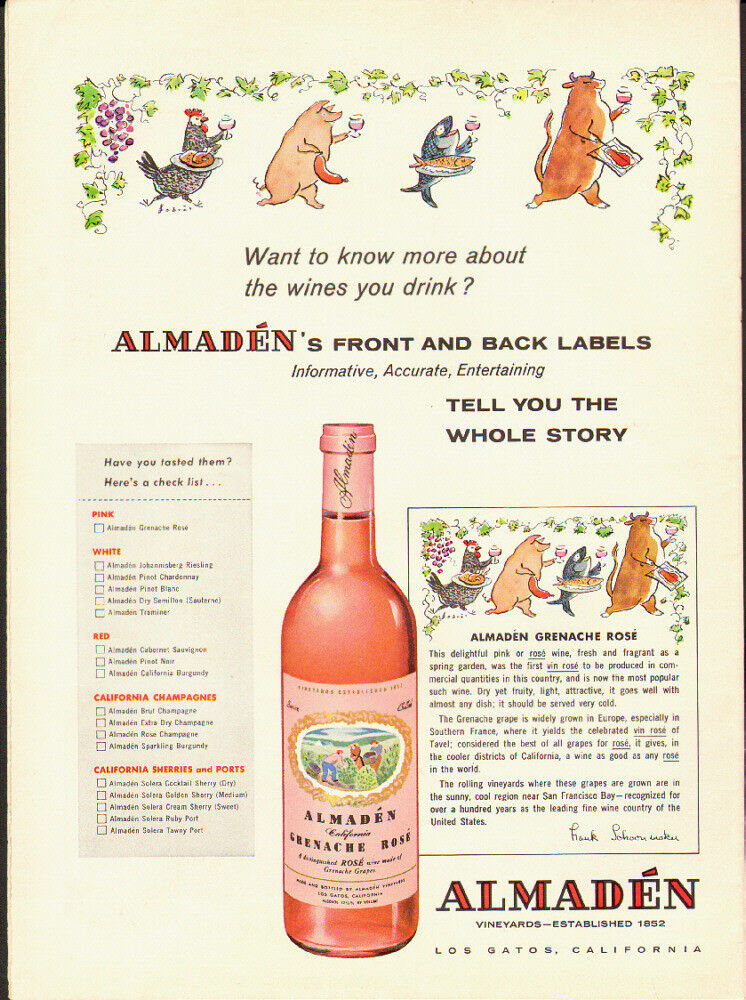This vintage advertisement for Almaden wine, rendered as a detailed drawing, features an array of whimsical animal characters promoting various wine varieties. At the top, a rooster carries a plate of chicken and a glass of wine, a pig holds a sausage and a glass, a gray fish bears a wine bottle and a fish on a platter, and a cow presents a glass of wine and a piece of steak on a grill. Above these lively illustrations, a header invites viewers to "Want to know more about the wines you drink? Almaden's front and back labels—informative, accurate, entertaining—tell you the whole story."

Below the animal ensemble, a comprehensive checklist categorizes Almaden's offerings into pink, white, and red wines, along with California Champagnes, Sherries, and Ports. Each variety's name is prominently prefixed with "Almaden," underscoring the brand’s extensive selection.

Prominently displayed in the center is a bottle of Almaden Grenache Rosé, adorned with a pink cap and label. Adjacent to the bottle, a detailed description lauds the wine as "fresh and fragrant as a spring garden," noting its historical significance as the first commercially produced rosé in the U.S. and its enduring popularity. The description highlights that this wine, made from Grenache grapes grown in both Europe and California’s cool regions near San Francisco Bay, is celebrated for its dry yet fruity taste and versatility with various dishes.

The advertisement is signed by Frank Schoonmaker, and the bottom right-hand corner of the image proudly declares "Almaden Vineyards, established 1852, Los Gatos, California."